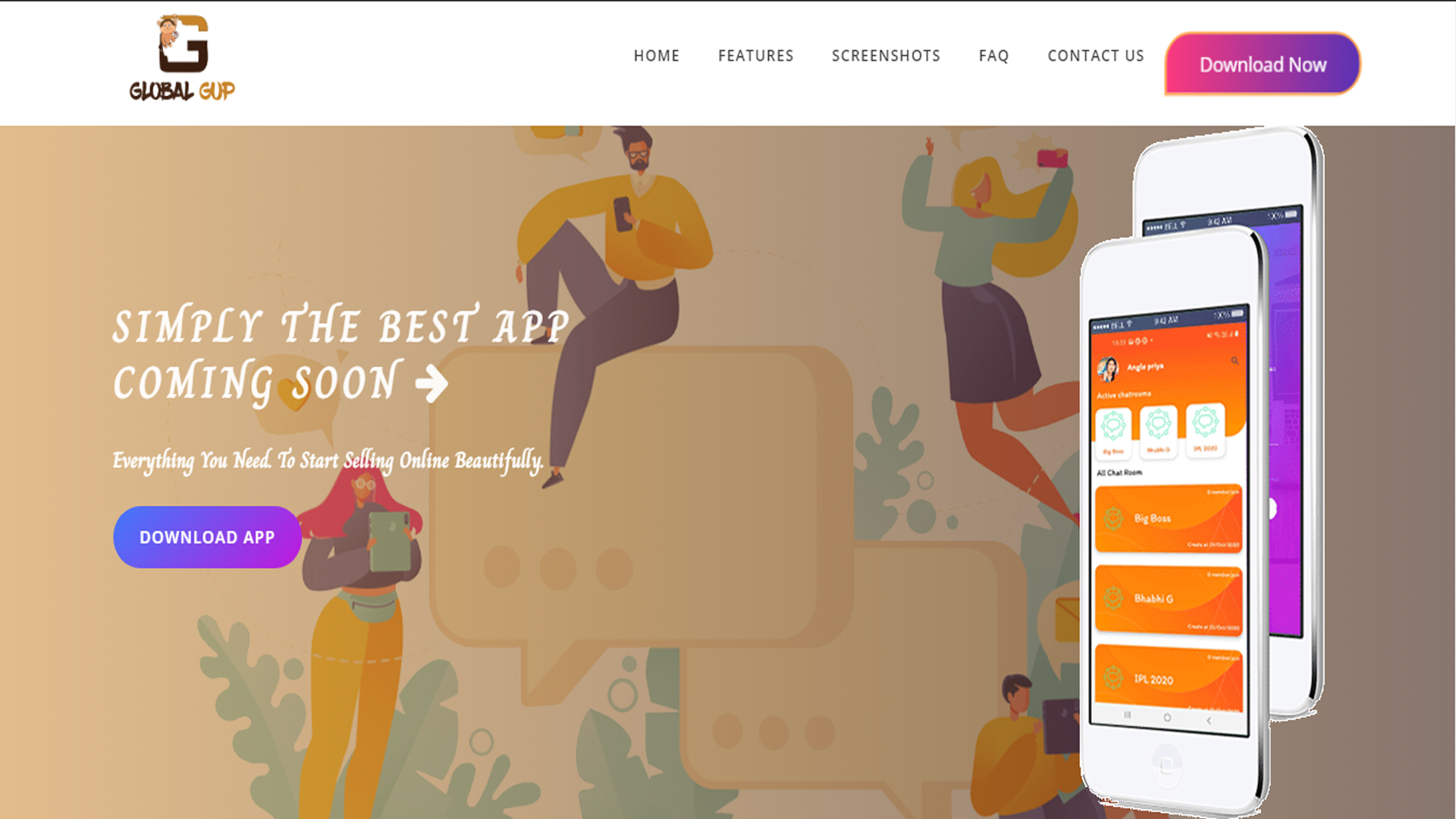The image showcases a website called "Global GUP," identifiable by a prominent 'G' insignia. The website's design is sleek, with a black bottom half and a tan top half. A white navigation bar at the top contains menu options: Home, Features, Screenshots, FAQ, and Contact Us, alongside a colorful 'Download Now' button outlined in orange with a gradient fill of purple, pink, and red.

Below the navigation bar, there's a tan-colored information box that prominently features the message "Simply the best app coming soon" in elegant, decorative typography. Adjacent to this message is a white arrow pointing to the right.

The right section of the webpage features an image of two white smartphones, one slightly behind the other, displaying app screens. The background includes illustrations of people engaging with their devices, with exaggerated, whimsical proportions. One character, a guy with a small head and an oversized body, is sitting on a message icon. Another character is a girl with blonde hair, depicted jumping with her phone and characterized by disproportionately large legs and buttocks but a smaller upper body. A red-haired girl, also with an exaggerated lower half, holds an iPad. There is an additional male figure below, barely visible, holding a computer.

The website prominently displays a call to action with the text "Everything you need to start selling online beautifully" followed by a 'Download App' prompt, which is highlighted in a purplish color.